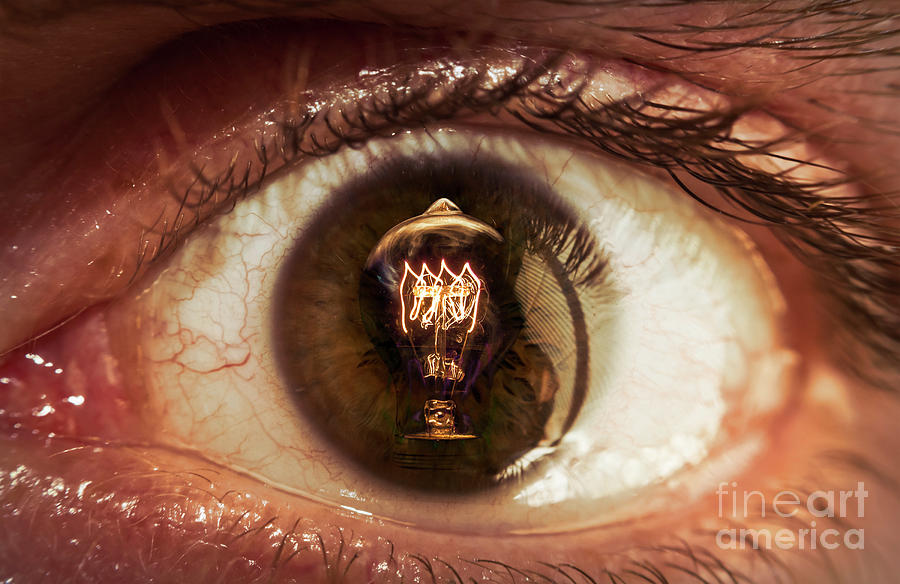The image is a highly detailed close-up photo of a human eye, with a strong focus on the iris and surrounding elements. The eye appears bloodshot, with numerous red vessels visible in the whites, giving it an unhealthy, glistening appearance. The iris is a blend of green and hazel hues, while the pupil is artistically replaced with an illuminated Edison light bulb, revealing intricate, glowing filaments that mimic electrical wires. The upper and lower eyelids, adorned with eyelashes, frame the eye, and the corner and edges of the eye appear moist, enhanced by small, pinkish water drops. In the bottom right corner of the image, the "Fine Art America" logo is subtly placed, serving as a watermark. This collage of elements creates a striking and imaginative visual effect.